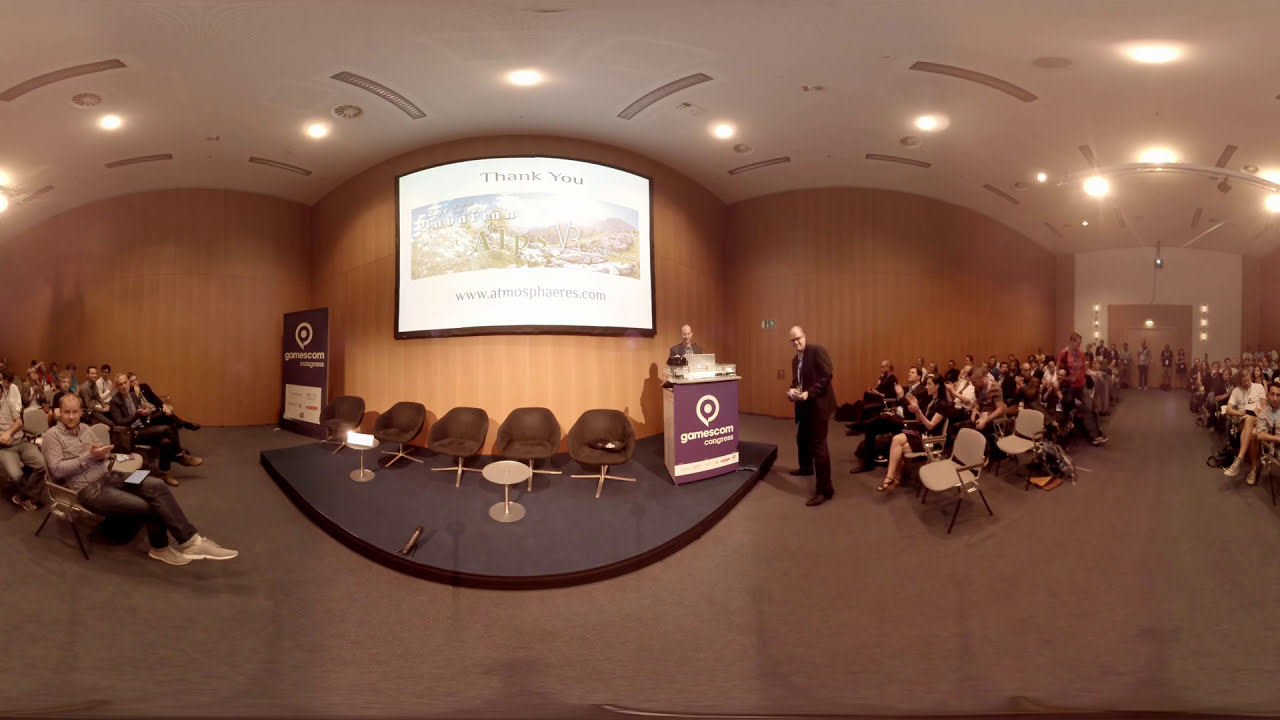The image depicts an indoor professional conference setting. At the forefront, there is a man standing at a podium with a white logo resembling a bullseye and some text that likely reads "games.com" or "games cam". Another man in a black suit with glasses stands next to him, while a man in a gray suit is also present. The stage has five empty dark brown or possibly black chairs. Behind the podium, a pull-down projection screen displays a "Thank you" message, with a background image of the outdoors and the website www.atmospheres.com. The audience, situated in gray or tan chairs, is divided by a central aisle leading to a set of open doors. The room features white walls and ceiling with lights, vents, and likely speakers, and a gray floor. The attendees appear engaged, some taking pictures and listening attentively to the presenter.